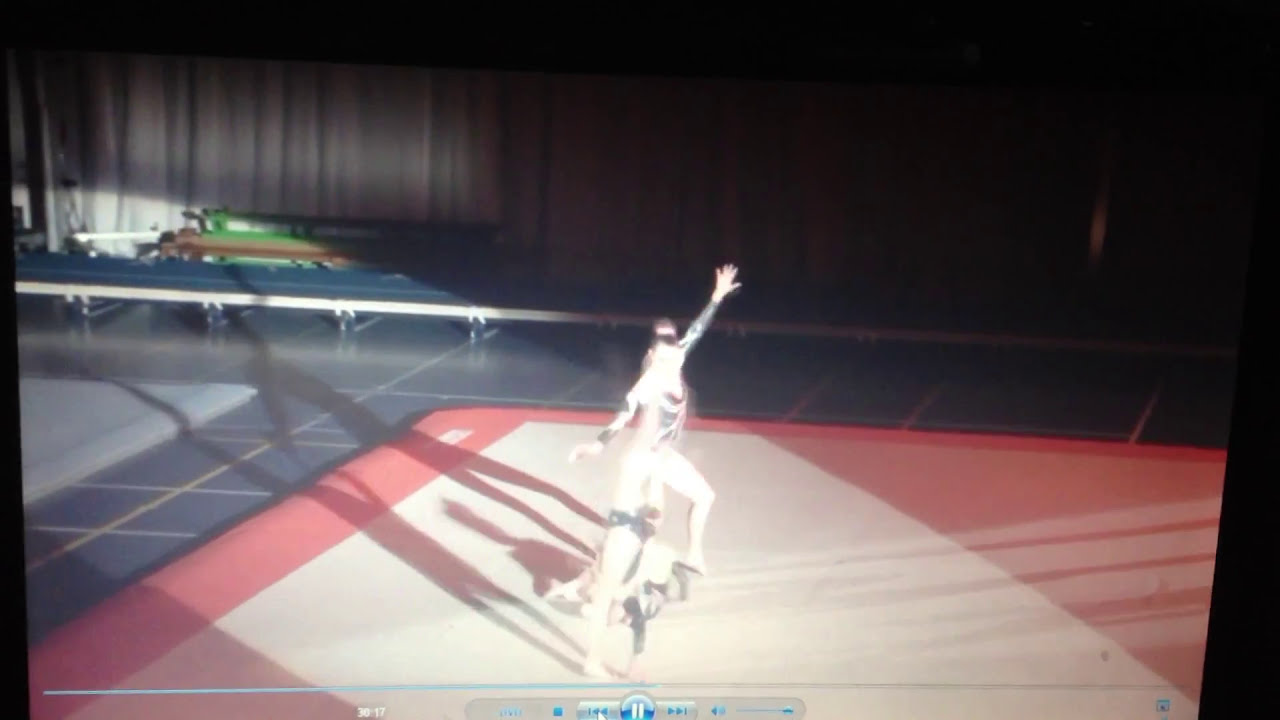The image is a photograph of a computer monitor showing a video playback in the Windows Media Player app. The video depicts a performance, potentially a gymnastics or circus act, featuring at least two acrobatic performers on a large red and white mat. The scene is heavily illuminated, causing the performers to appear almost whited out, making their features difficult to discern. The well-lit performers, who seem to be light-skinned and include two females, are engaged in dynamic poses; one is wearing a black leotard with one arm extended above her head, the other arm down, and one leg bent with the toe pointed on the ground. The second performer seems to be mid-cartwheel, and the shadows cast suggest there may be a third performer. The background features dark curtains and what appears to be a balance beam. At the bottom of the screen, typical media player controls including play, pause, fast-forward, and volume adjustment are visible, along with a progress bar indicating the video's timeline.